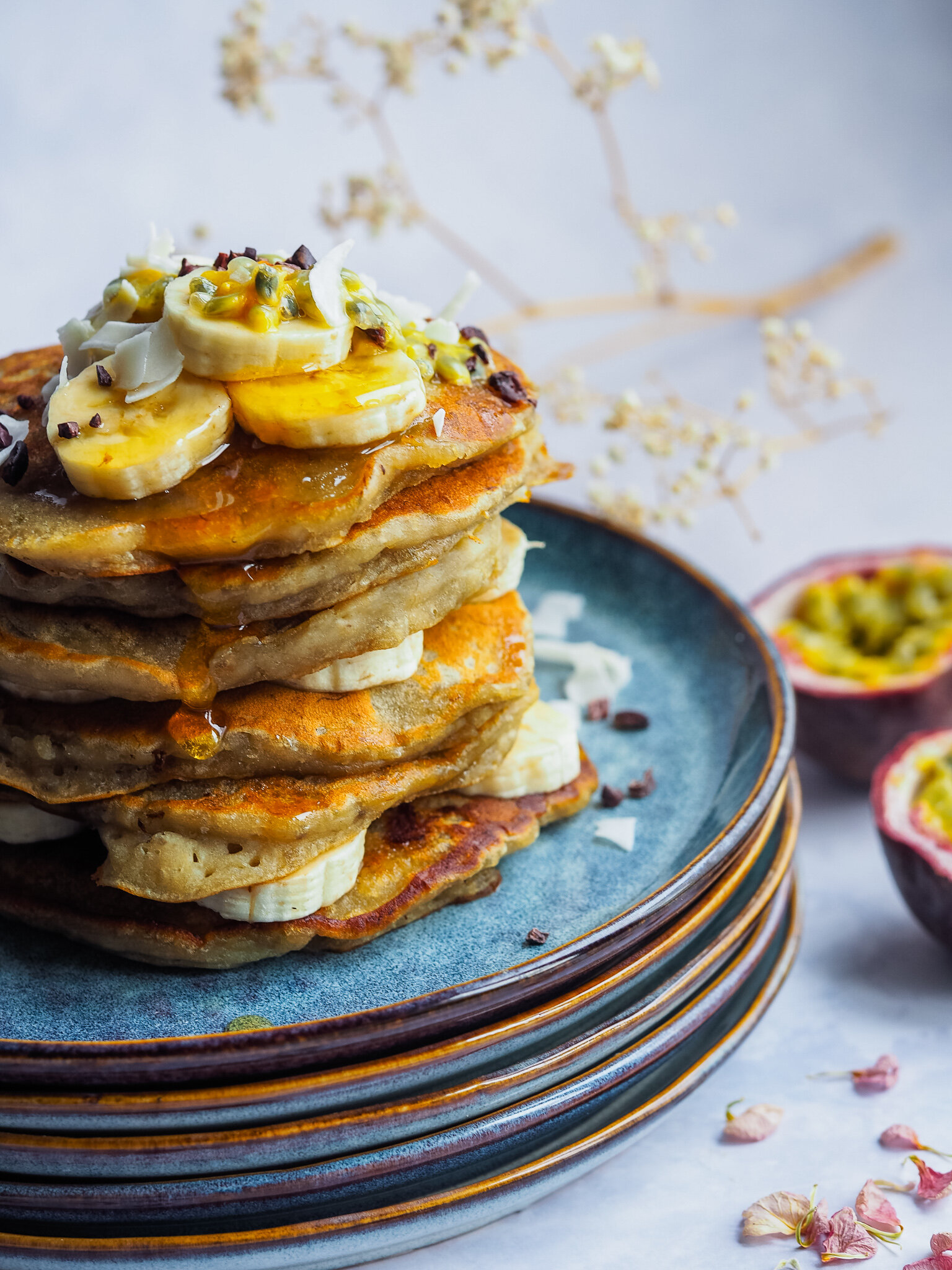This photograph captures a sumptuous stack of pancakes meticulously layered with slices of bananas between them. The tower of approximately seven fluffy, seared pancakes varies in shades from light brown to dark brown. Nestled between almost every pancake are slices of banana, offering a delightful contrast. The pancakes are generously drizzled with caramel-colored syrup, cascading down the sides, adding to their mouthwatering appeal. 

Adding to the visual and textural feast, the pancakes are garnished with dark chocolate chips and a sprinkling of fine white shavings, potentially coconut flakes or thinly shaved butter. The topmost pancake features an additional small stack of sliced bananas, completing the decadent presentation.

These delicious pancakes are presented on a beautifully decorated, bluish-green, ceramic plate with white patterns and a touch of gold paint around the perimeter. This topmost plate sits on a stack of three or four similarly styled plates, enhancing the visual layers of the presentation.

In the background, on the right side, there is a cut-open passion fruit revealing its vibrant yellow-green seeds against a red outer shell, identifiable by its distinctive look. Additionally, a few delicate flower petals can be seen scattered at the bottom right corner on a grayish surface, with a stem of white flowers subtly peeking from behind, adding a touch of natural elegance to the scene.